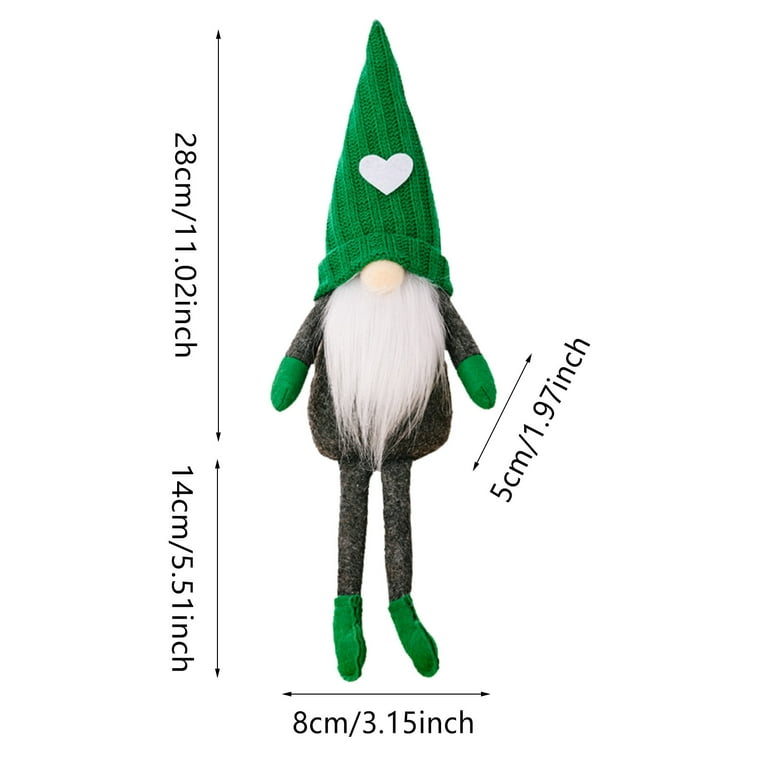The image features a detailed product shot of a Swedish Dwarf figurine, often referred to as a toy goblin, prominently displayed on what appears to be a retail website. This whimsical figure is characterized by its large green hat adorned with a white heart, which drapes over its eyes, revealing only its prominent button nose and lush white beard. The figurine’s attire comprises a gray outfit made of cloth, along with coordinating green hands and boots. Its short arms contrast with the long, dangling legs, adding to its quaint appearance. Dimensions are clearly marked beside the figure; the overall height is approximately 32 cm (11 inches), with the top half measuring 28 cm (11 inches) from head to waist and the bottom half from waist to toe at 14 cm (5.5 inches), a width of 8 cm (3.15 inches), and a waist width of about 5 cm (2 inches). The background of the image is plain, emphasizing the dwarf and its whimsical, charming details for potential customers.